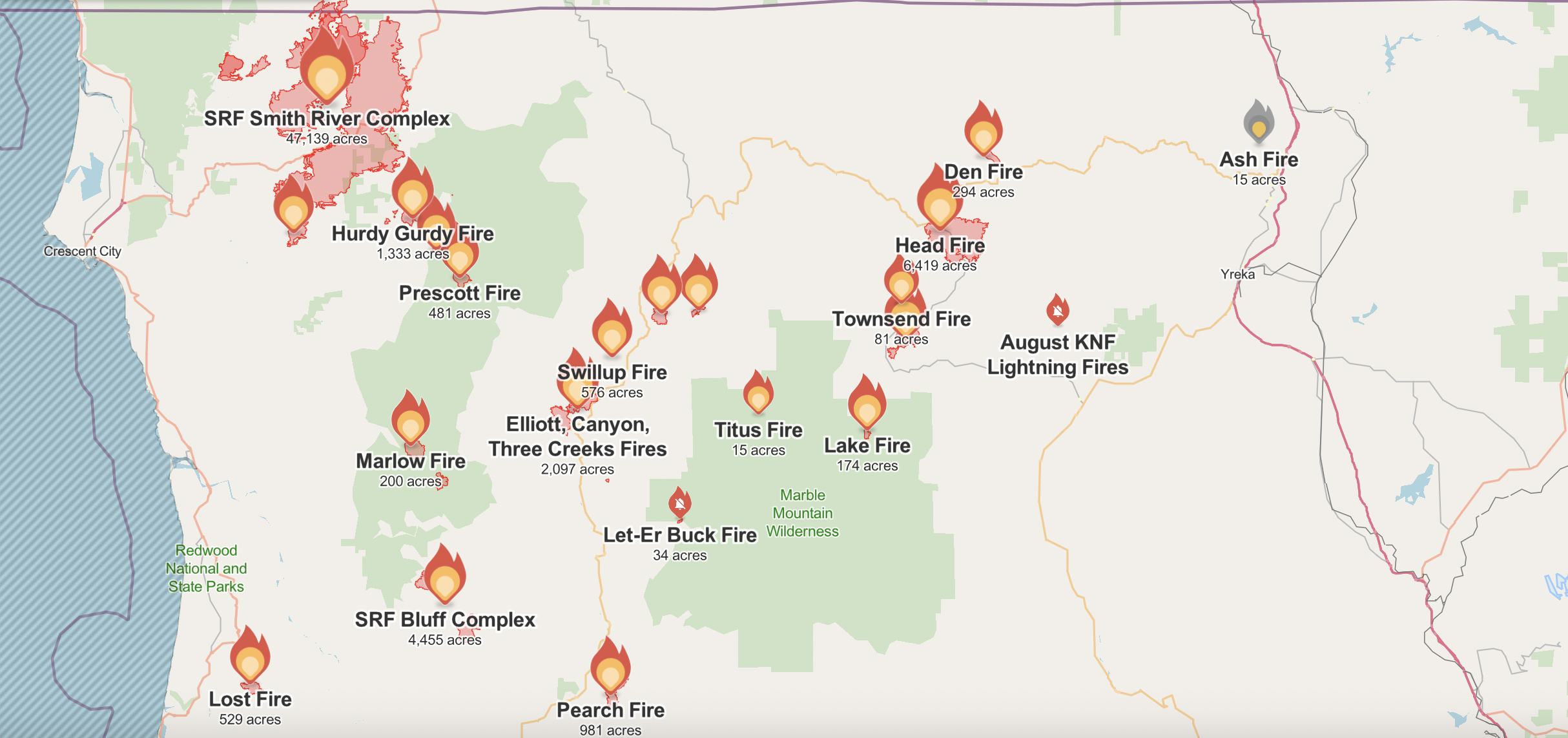This detailed image is a close-up portion of a map, specifically of Redwood National and State Parks, with land depicted in white and green primarily on the right side and water in blue on the left. The map is densely populated with flame icons in light orange, dark orange, and red, representing wildfires, with about two dozen icons varying in size to indicate the severity of each fire. The icons are not randomly placed; they cluster particularly towards the top left, where some regions are outlined in red and labeled with specific fire names like Townsend Fire, Lightning Fires, Perch Fire, and Den Fire. The map also notes the acreage affected, such as Den Fire at 294 acres and Ash Fire at 15 acres. Additionally, the map features labels, wilderness areas, and indications of rivers, particularly visible on the right side as thin blue lines, along with roads and other geographical details, effectively mapping out the wildfire locations across the park area.